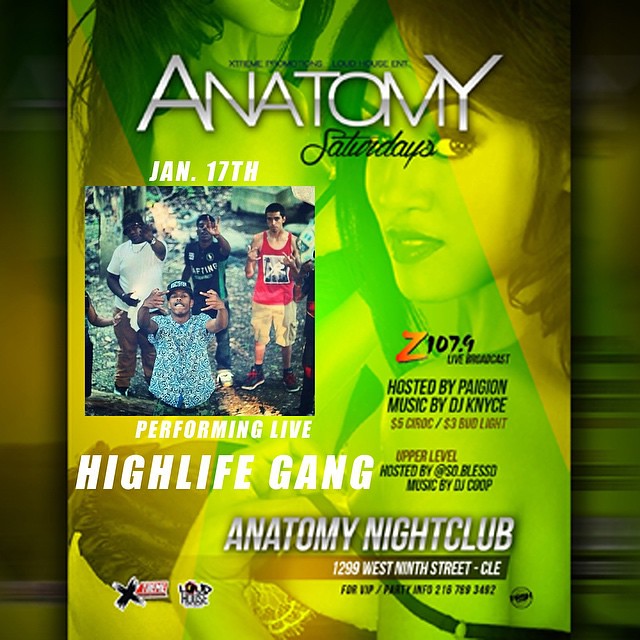The promotional flyer for "Anatomy Saturdays" features a vibrant green and yellow textured background, overlaid with images of stylishly dressed African-American women. The top of the flyer prominently displays "ANATOMY" in white, chrome-like font and “Saturdays” in black cursive text. Above "ANATOMY", there is some small, illegible black font text. The event date "Jan. 17th" is clearly positioned in the center, below which is a photo of four men—three African-American and one of Mexican descent—casually posing with sparklers and making hand gestures. The middle left of the flyer contains the text "Performing Live High Life Gang" in white font. 

To the middle right, details about a live broadcast by Z107.9 in black font are featured, including mentions of the hosts: "Hosted by Pygon," "Music by DJ KNYCE," "$5 Ciroc," and "$3 Bud Light." Additionally, it includes "Upper Level" in reddish font, and "Hosted by @So.Blessed," "Music by DJ Coop" in black font.

The bottom section provides essential venue information: “Anatomy Nightclub, 1299 West 9th Street - CLE” in white font, with contact information for VIP/party inquiries (216-788-3492) in smaller black font. Company logos for Extreme and Loud House also appear in this segment, adding a finishing touch to the flyer.